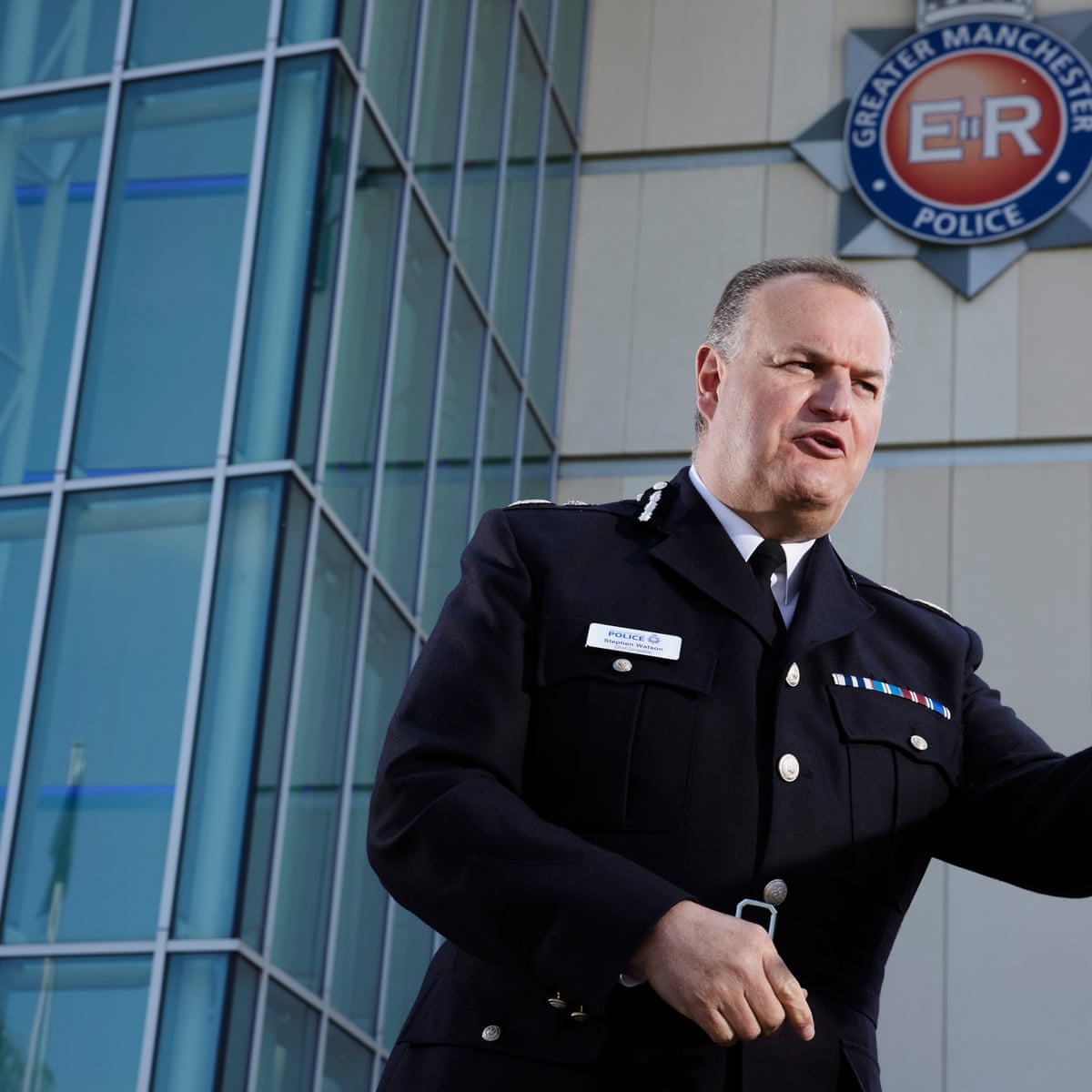This is a highly detailed color photograph of a Caucasian man, likely between 50 and 65 years old, who appears to be a decorated police officer. He is standing in front of a modern police station characterized by concrete elements and glass panes with metal frames. The building prominently displays a circular logo with the inscription "Greater Manchester Police" and the letters "ER" within it.

The officer is dressed in an official black police uniform that includes a name tag on the right breast pocket, two buttoned breast pockets, silver buttons down the center, a belt around the waist, and a white shirt underneath. His uniform is adorned with various colorful threads and awards, highlighting his decorated status.

The man is captured mid-speech and is gesturing with his hand, possibly giving directions or emphasizing a point. Despite the photograph's professional lighting, the resolution makes the name on his badge indiscernible. This staged portrait, with its detailed setting and clear depiction of the officer in his formal attire, underscores the significance and professionalism of his role in the Greater Manchester Police.